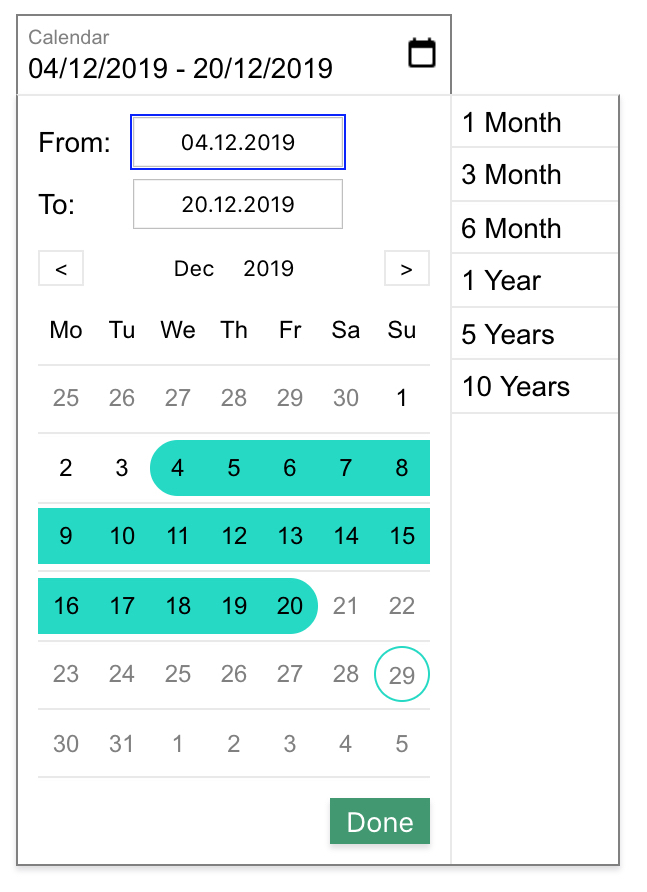Here is a detailed and cleaned-up caption for the image:

"A screenshot of a calendar application interface displaying a date range selection. At the top, there is a grey header with the word 'Calendar', followed by the date range '04-12-2019 - 20-12-2019', and a small black calendar icon to the right. The background is white with a black border framing the application. Below, a date selection section highlights the range '04.12.2019' to '20.12.2019' within a blue-bordered white box. Navigation arrows flanking 'December 2019' are present above the day headers: Monday through Sunday. The dates within the selected range (04 to 20) are highlighted in blue, while the 29th is circled in blue. A green 'Done' button is located at the bottom. On the right side, a sidebar menu lists time intervals: 1 month, 3 months, 6 months, 1 year, 5 years, and 10 years."